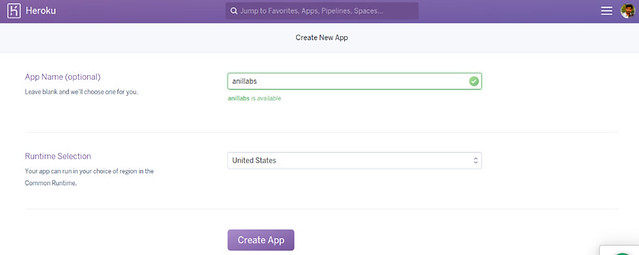The Heroku website features a primarily white page with a light to medium purple top bar. On the left side of this bar, "Heroku" is prominently displayed in white text against the purple background. Centrally located on the bar are navigation options: "Jump to Favorites," "Apps," "Pipelines," and "Spaces," each separated by commas. To the right, three horizontal lines are displayed, next to which is an image icon.

Beneath the purple bar, the main content area has a white background. At the top center of this section, the text "Create new app" is displayed in black. Below this header, the first line reads "App name (optional)" on the left side. To the right of this line, a green rectangular highlight contains the text, which appears to say "anneal labs," though the exact wording is not entirely clear.